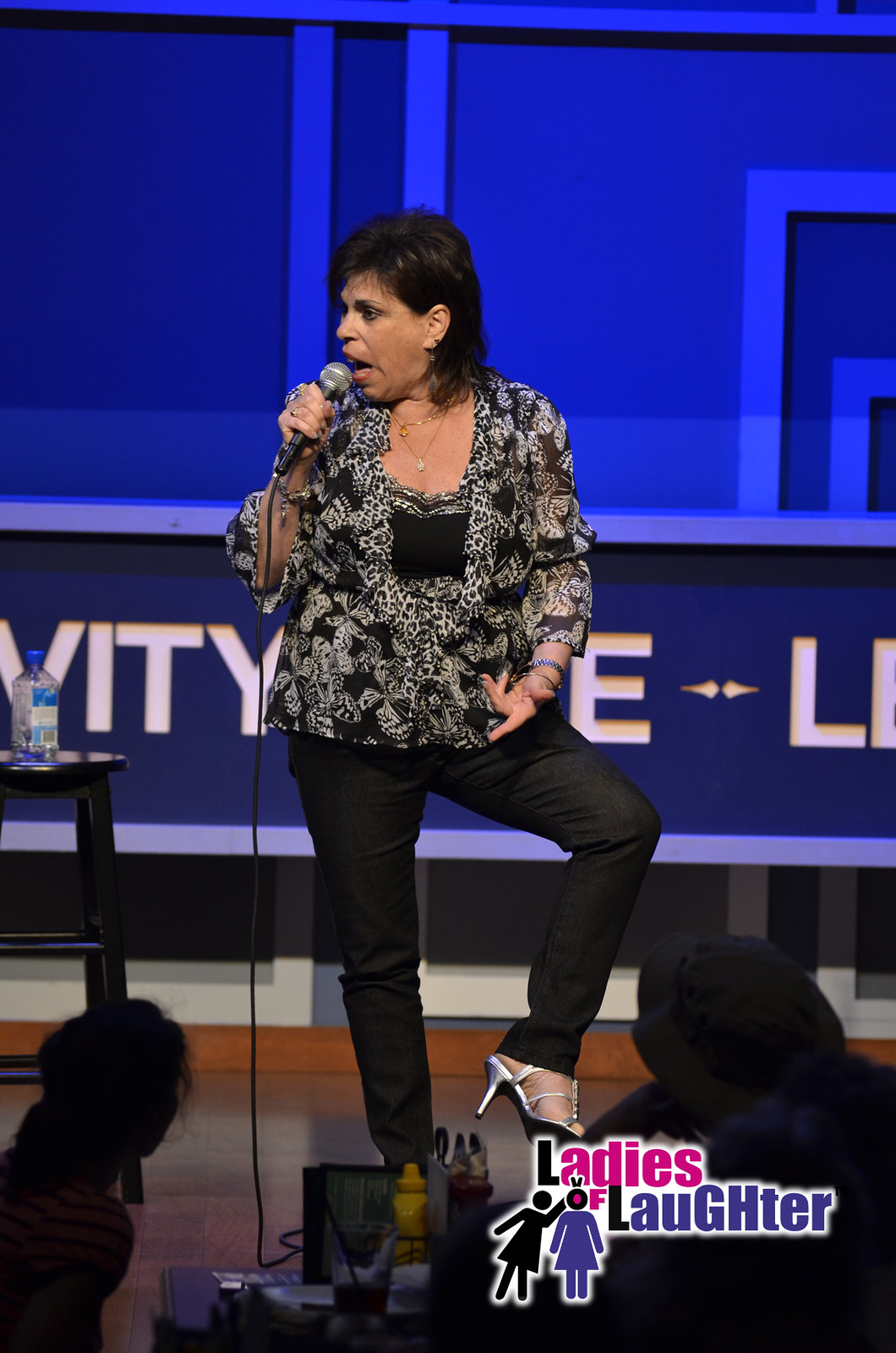The photograph captures a female stand-up comedian mid-performance on a wooden stage, backed by a blue curtain adorned with partially obscured white letters that include "V-I-T-Y." The comedian, with short dark hair, is animatedly speaking into a microphone held in her right hand, while her left hand gestures expressively, emphasizing her points. She is dressed in a stylish black and gray patterned blouse, black pants, and striking silver high heels, with one knee playfully lifted off the ground. A black bar stool nearby hosts a water bottle with a blue cap. In the foreground, silhouettes of audience members seated at tables can be seen, with bottles of mustard and ketchup adding a casual dining element to the scene. The bottom right corner of the image features the "Ladies of Laughter" logo, styled in black, pink, and purple fonts, accompanied by two outlines of women, one appearing to reach towards or punch the other.